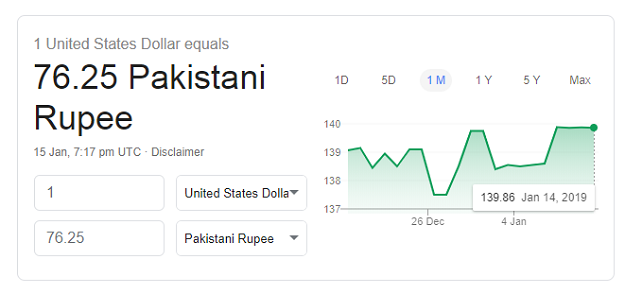A screenshot captures a currency conversion tool on a white background, bordered by a thin gray line. In the top left corner, gray font text indicates, "1 United States dollar equals," followed by a large, bold black font showing, "76.25 Pakistani Rupee." Directly beneath, gray font states the date and time: "15 Jan 7:17 p.m. UTC," along with a "Disclaimer" note.

The tool features a dropdown menu with two boxes labeled "United States dollar" and "Pakistani rupee," allowing users to input the amount they wish to convert between the currencies.

On the right side of the rectangle, a green line graph is displayed, illustrating the fluctuation in the exchange rate between the two currencies. The graph shows a significant dip on December 26th, followed by a sharp rise a few days later. The highlighted date on the chart is January 14, 2019, indicating the most recent exchange rate change.

Overall, the interface provides a visual and numerical representation of currency conversion and exchange rate trends between the US dollar and the Pakistani rupee.